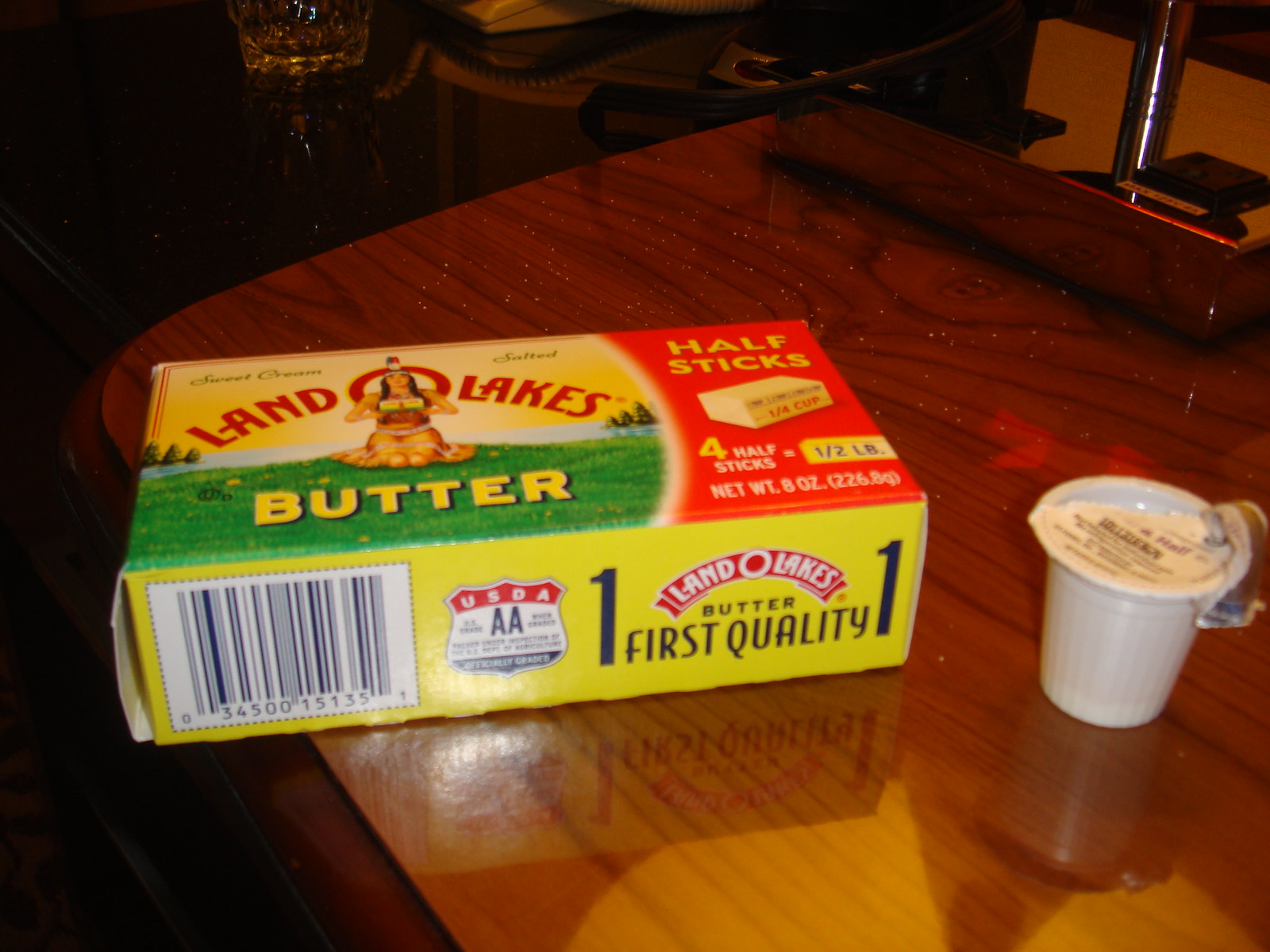This is an indoor color photograph featuring a detailed arrangement of items on a wooden tabletop with a glossy black border. Prominently displayed is a rectangular, yellow carton of Land O'Lakes butter featuring a picture of a kneeling Native American woman in a grassy meadow. The carton specifies that it contains four half sticks of butter, totaling a half pound (8 ounces or 226.8 grams), and includes a barcode and a USDA label marking it as "First Quality". To the right of this is a white, single-use coffee creamer container that appears to have been torn open. At the top of the image, a clear glass is partially visible. Additionally, a corded landline phone and various indistinct objects, including what may be a plaque and a silver pen, are scattered along the table's border.